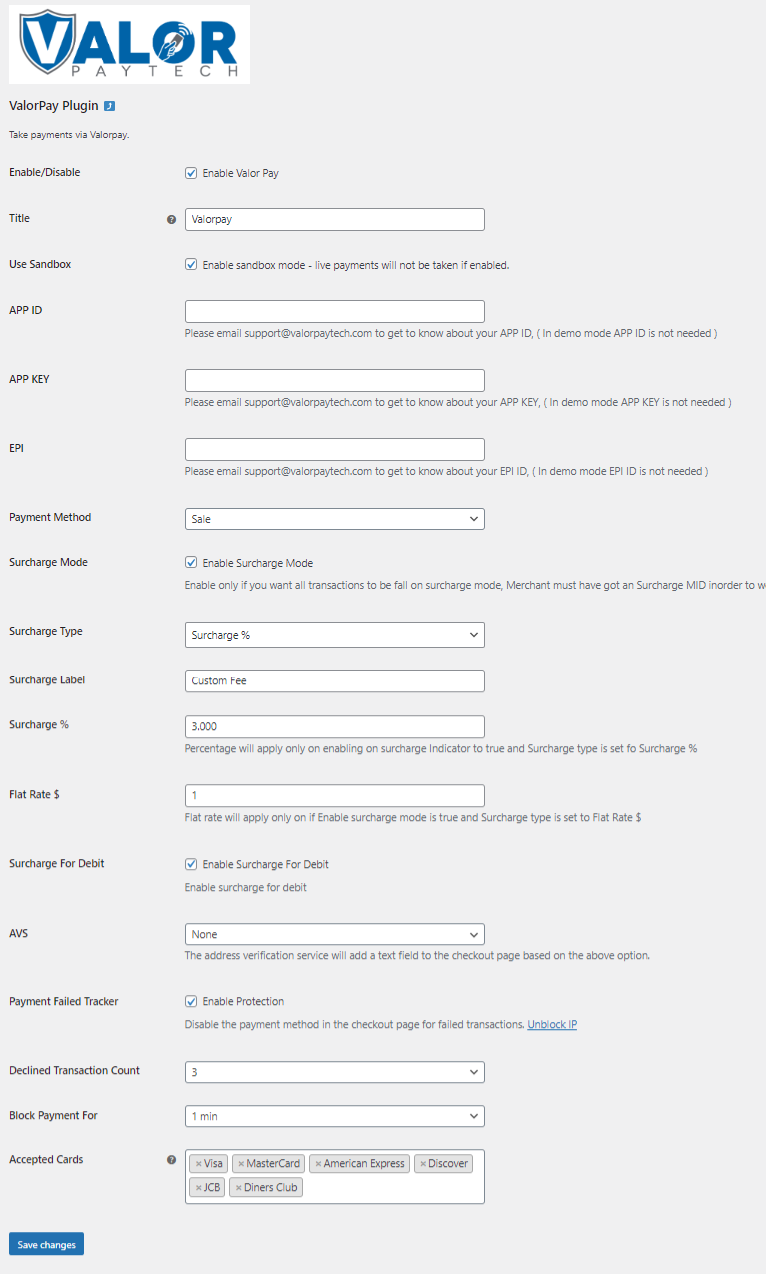This screenshot captures the interface of a computer program, specifically for Valor Paytech. The page features a gray background with various text entries and white input boxes for user configuration.

In the top-left corner, the Valor Paytech logo, which includes a badge around the letter "V," is clearly visible in a small white box. Beneath the logo, the text "Valor Pay Plugin" and options for toggling settings like "Take Payments" (with an enable/disable checkbox) are displayed.

Key configuration options are listed on this page, including:
- Title: "Valor Pay"
- "Use Sandbox" with an explanatory note: "You can click this to enable Sandbox Mode. Live Payments will not be taken if enabled."

Further down, fields for entering "App ID," "App Key," and selecting from a dropdown box labeled "Payment Method" (currently set to "Sale," with other possible choices) are available. 

Additional settings include:
- "Surcharge Mode" (with an enable checkbox)
- "Surcharge Type" with a dropdown displaying "Surcharge Percent"
- Label fields like "Surcharge Label," "Custom Fee," "Surcharge Percent," and "Flat Rate Dollar"
- Specific options like "Surcharge for Debit" and "AVS"

For tracking and security, there's 
- "Payment Failed Tracker"
- "Decline Transaction Count" (set to 3)
- "Block Payment for" (set to 1 minute)

Lastly, the "Accepted Cards" section lists the supported payment cards: Visa, MasterCard, American Express, Discover, JCB, and Diner's Club.